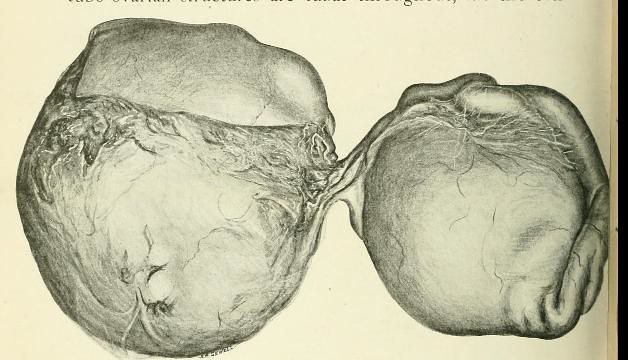This is a nearly black-and-white photograph featuring what appears to be a drawing or sketch of two round, bulbous masses, resembling human organs. The background is a faded yellow, akin to an aged paper page from a book, and there is no clear identifying information or labels on the image. Both masses, which are connected at the center by tissue or nerve-like structures, have a detailed, veiny appearance, suggesting they could be fibroids, tumors, or even a crude depiction of lungs or other organs. The mass on the left is noticeably larger than the one on the right. The image is approximately five by four inches in size, and there is partial, cut-off text along the top edge of the photograph.